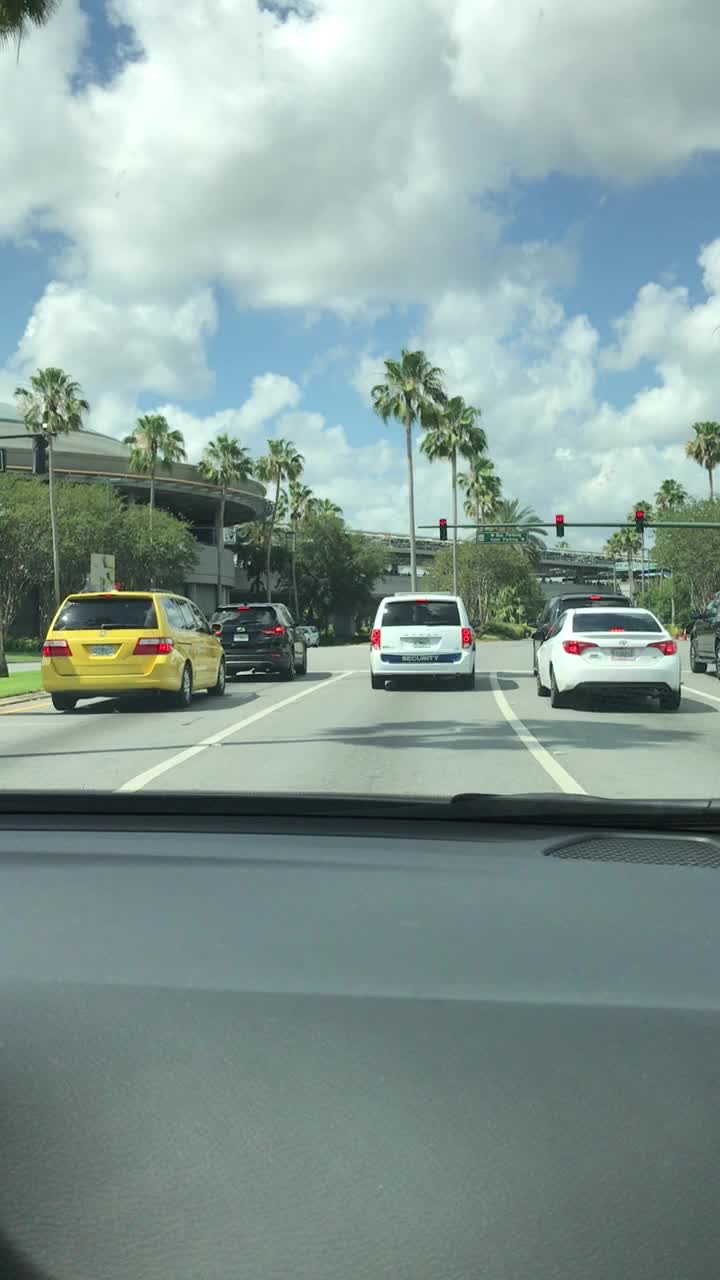The image is captured from the inside of a car, presenting a first-person perspective through the front windshield. The photograph has a vertical orientation, emphasizing the view from the dashboard to the distance ahead. Within the car, we can observe the dashboard prominently, including the top right corner speaker grille and the sealing edge around the window. The windshield wipers are also visible.

Outside the car, there is a gap of approximately five to seven meters before we reach the rear of a white car that is halted at a red traffic light. This car is positioned in one of four lanes, all directed in the same way. Beside it, on the left and right, there are three additional lanes stocked with vehicles also waiting at the stoplight.

On the far left, beyond the leftmost lane, a grassy median divides the traffic directions. This median is lined with tall, stately palm trees that extend into the distance, creating a picturesque barrier. Overhead, the sky is a mix of light clouds with patches of blue, indicating a relatively clear day despite the clouds. The overall scene conveys a typical urban traffic moment under mildly cloudy but bright conditions.